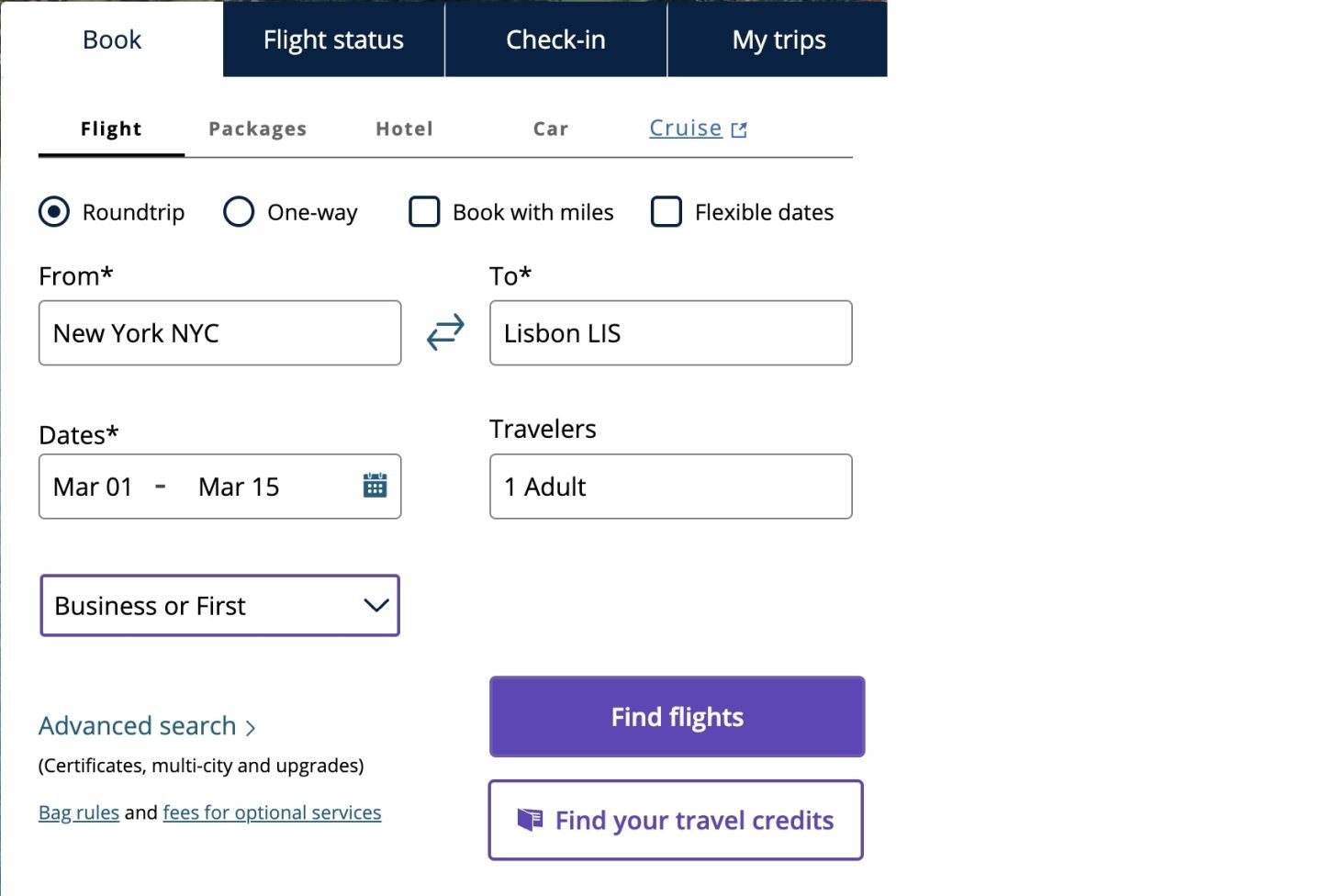Displayed is the booking interface of a travel website, featuring four primary tabs at the top: "Book" (selected), "Flight Status", "Check-In", and "My Trips". Below the "Book" tab are options specific to booking: "Flight" (currently selected), "Packages", "Hotel", "Car", and "Cruise". 

In the "Flight" booking section, users can choose between "Round Trip" and "One-Way" flights, as well as options to "Book with Miles" and specify "Flexible Dates." The "Round Trip" option is currently selected, with the "From" field set to New York and the "To" field set to Lisbon. The travel dates are specified as March 1st to March 15th, though these can be altered as needed. The number of travelers is set to one adult, and the travel class is set to "Business or First Class".

There is an "Advanced Search" option for more customized queries. To the right of this section is a prominent purple button labeled "Find Flights", for initiating the search process. Below it is a white button with purple text reading "Find Your Travel Credits".